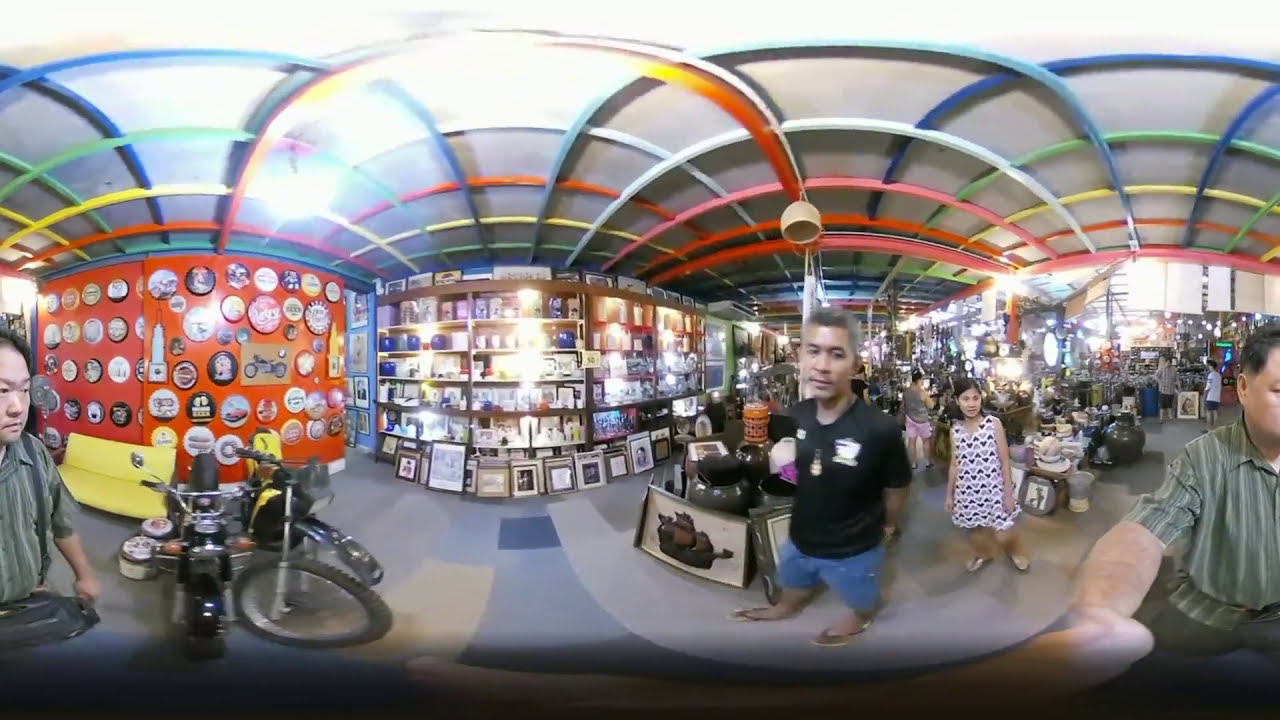This panoramic image depicts the inside of a large, old-fashioned store, possibly an antique or thrift shop, filled with a diverse array of items. Dominating the center back wall, a collection of framed pictures and prints are neatly displayed. The store's right side features assorted mirrors, lamps, and metallic pieces, while the left side is adorned with decorative plates and circular, bottle cap-like decorations. The floor is covered with an old carpet, enhancing the nostalgic ambiance suggestive of a 90s-era establishment. Down the middle aisle, a mix of motorcycles, vases, pots, and pans are seemingly scattered. The ceiling is notably colorful, designed with overlapping semicircles in reds, blues, whites, pinks, yellows, and greens, reminiscent of a fish scale pattern. Several casually-dressed Asian individuals, including a man in a black t-shirt and shorts, can be seen walking around the store, browsing the eclectic assortment of items, suggesting a lively, bustling atmosphere in what could be a souvenir or antique shop during the spring or summer.